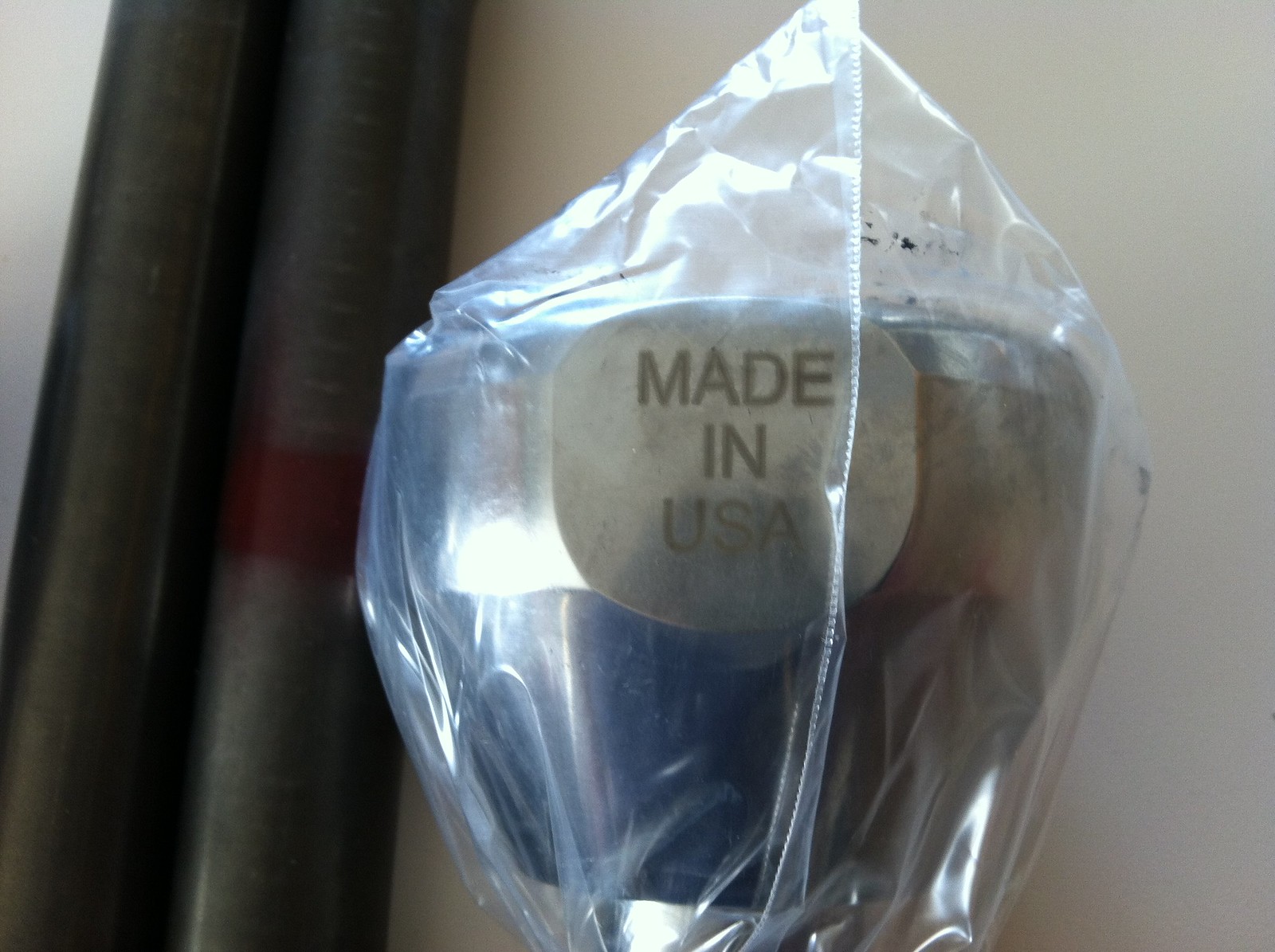The image depicts a small, clear plastic wrapper tightly encasing a silver and black, dome-shaped object. On the front of the object, there is a grey, slightly dirty patch bearing the inscription "Made in USA" in black, capitalized letters, with each word occupying its own line. The object itself has a wider, circular top that tapers down to a silver point at the bottom. The background features a tan-colored wall, with a black or grey curtain partially covering the left side of the photograph.